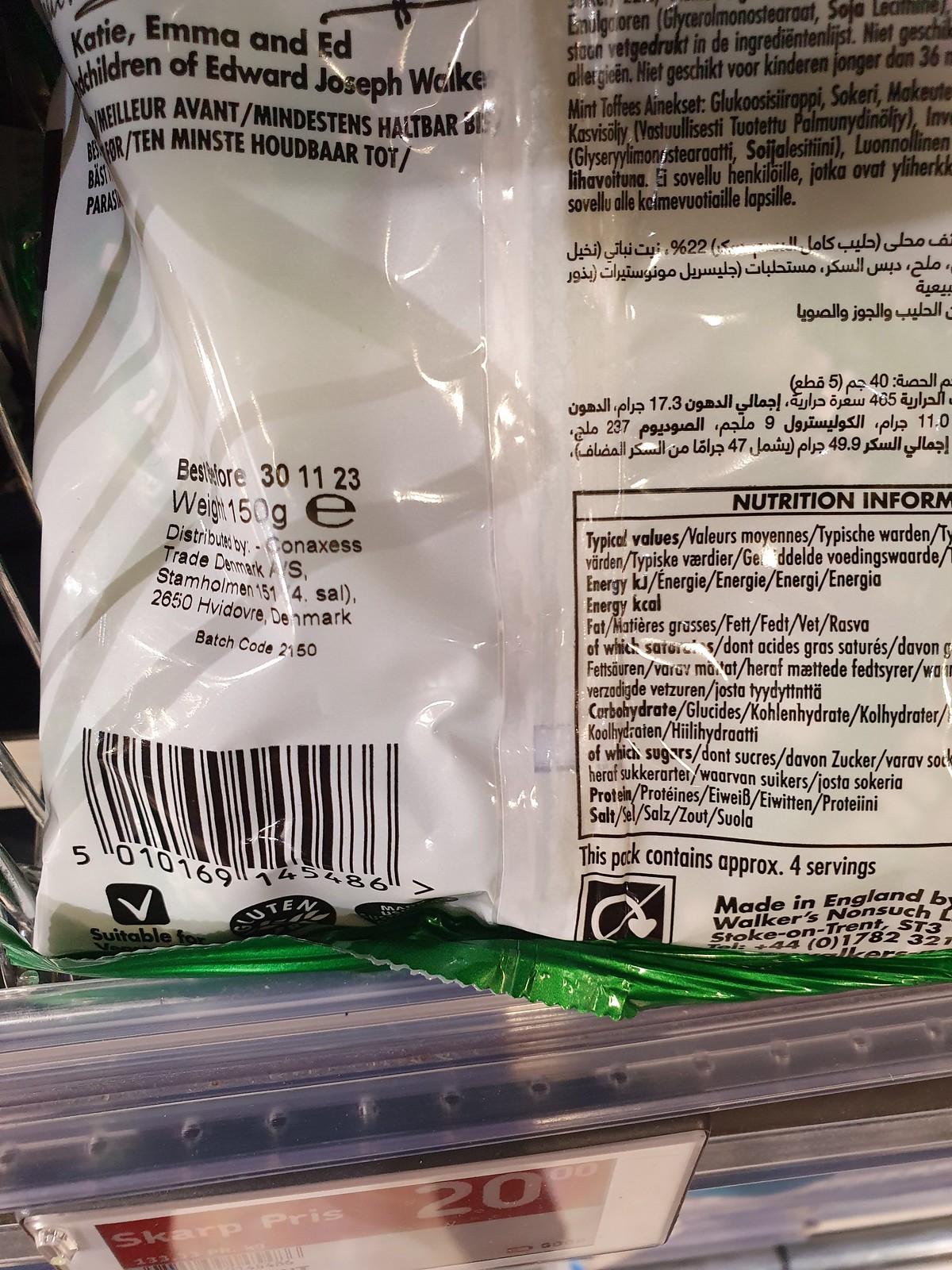This close-up photograph captures the detailed back side of a food package. The package itself is primarily white with black lettering, complemented by a green bottom section. Central to the layout is a dedication: "Katie, Emma, and Ed, children of Edward Joseph Wyken." Directly beneath this is a barcode. The package indicates that it contains a product weighing 150 grams and includes information about distribution with the trademark "Denmark, Stomholman." The batch code is listed as 2150. 

On the lower right side, it specifies that the contents provide four servings. The package's origin is noted with, "Made in England by Walker's Nonsuch, Stoke-on-Trent ST3," and a phone number is provided for further contact. Above the manufacturing information, a section is dedicated to the nutritional information of the product.